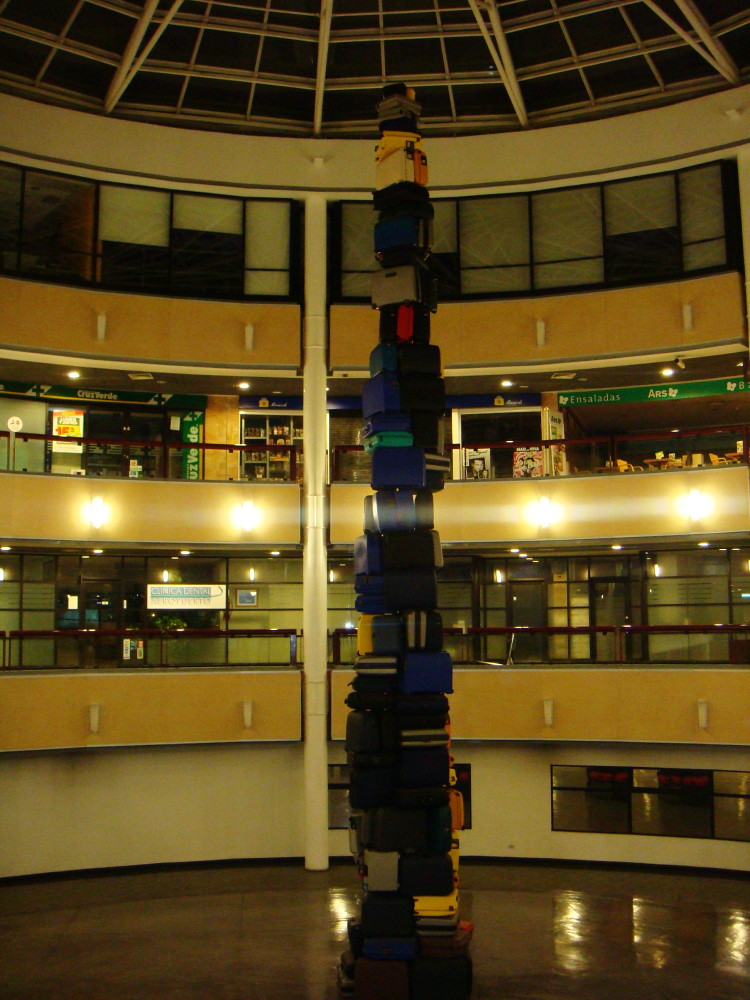The image depicts a color photograph of a large, round atrium, likely within a commercial building such as a mall, hotel, or airport. The atrium features a striking geometric glass dome roof with a grid pattern of white lines. Beneath this dome are three different levels. The top floor is lined with a series of windows equipped with both white and gray shutters, some raised to varying heights. On this level, a yellow partition is visible, contrasting with the building's otherwise subdued color palette.

The middle floor hosts a variety of elements, including a legible white sign displaying the words "ensaladas" and "ARS" on the right side near the ceiling. Below the sign are tables and chairs, suggesting the presence of a dining area or restaurant. A white entryway is seen on the left half, adjacent to what might be a storefront. Additional details on this floor include a yellow door, a green banner, and a blue banner adorned with plus signs on a white background.

The bottom floor primarily features windows and has a white banner with a blue graphic and unreadable text. There is another yellow divider here, along with a mix of windows or possibly mirrors on the right side.

Centrally located in the atrium stands a towering, thin pillar composed of variously colored suitcases stacked nearly four stories high, resembling a Christmas tree shape. This modern art installation adds a unique aesthetic to the space. Reflecting the light from above, the highly polished wooden floor enhances the overall ambiance of the atrium.